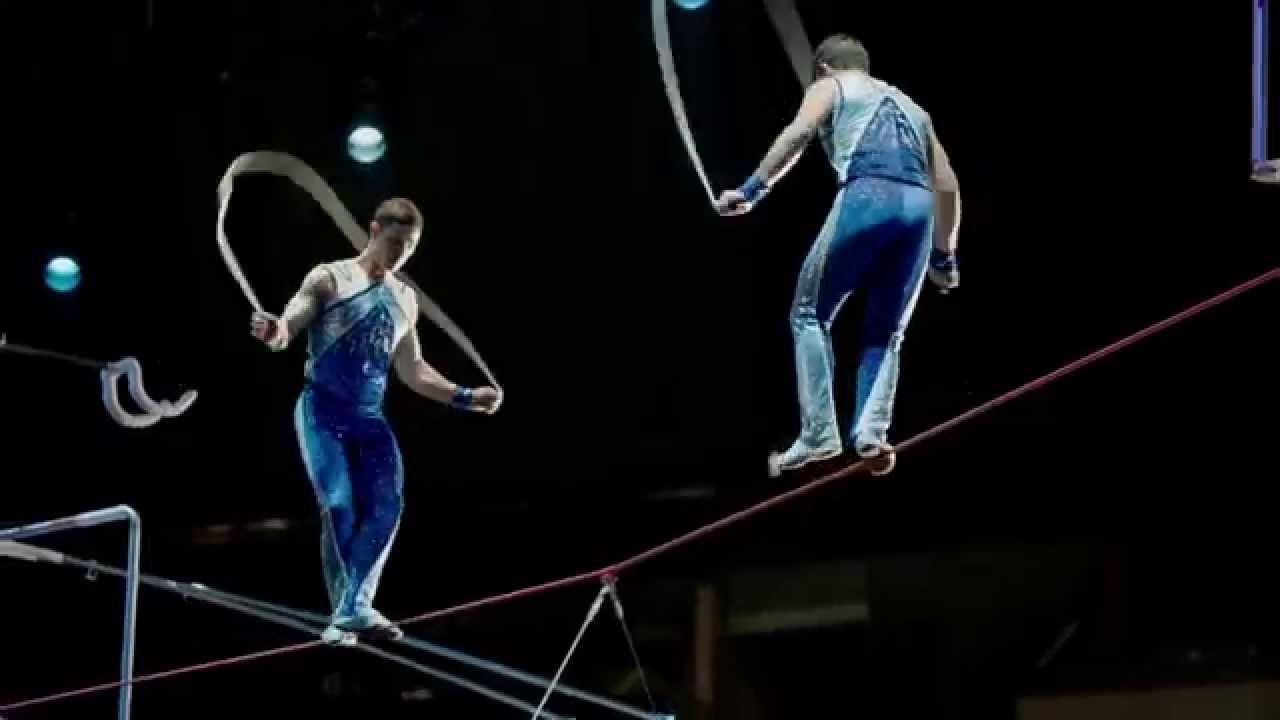The photograph captures an exhilarating circus act featuring two muscular male acrobats, both of whom appear to be Caucasian, balancing on a slender, red tightrope. The performers, clad in coordinated blue and white gymnast jumpsuits that include vests and pants, are captured mid-action in an intense spotlight against a completely black background. Each acrobat grasps a jump rope, which appears blurred from motion, indicating the dynamic nature of the stunt. The image is an aerial shot taken from the ground, emphasizing the height and skill involved. One acrobat is in the process of jumping, with his left foot raised and his back facing the camera, while the other stands with both feet on the tightrope, looking downward in concentration. Additional circus equipment and faint spotlights are visible in the background, enriching the scene with the atmosphere of a lively circus performance.